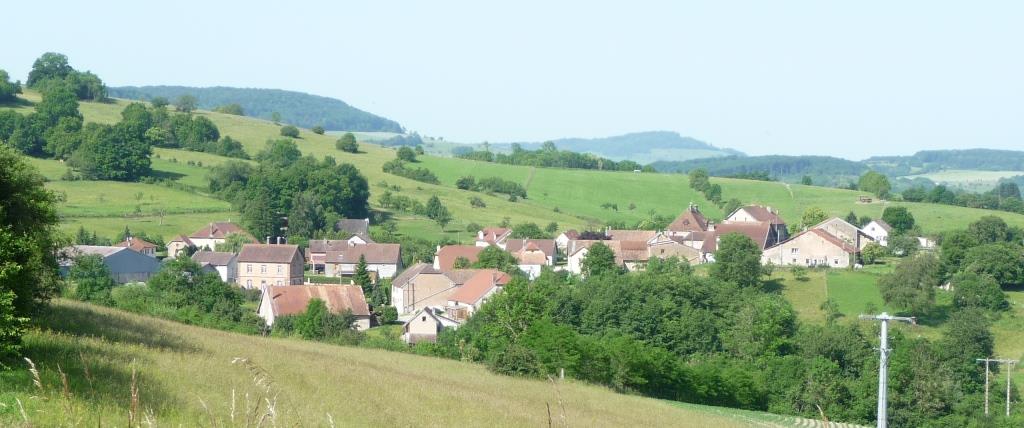The image captures a serene, panoramic countryside scene with rolling, grassy hills extending into the distance. In the foreground, a lush, green hill gently slopes down to a small village nestled between more hills. The village features a cluster of around 15 houses, most of which are two stories tall with white siding and light brown or light red roofs, giving the area a somewhat modern appearance. Scattered trees add bursts of greenery throughout the village and its surrounding landscape. Telephone poles are noticeable along the right side and within the village itself. As the hills rise again in the background, they eventually give way to far-off mountains, shrouded in a light, hazy fog. The image, taken from an elevated viewpoint, showcases the tranquility and beauty of a summer or spring day under a clear blue sky.